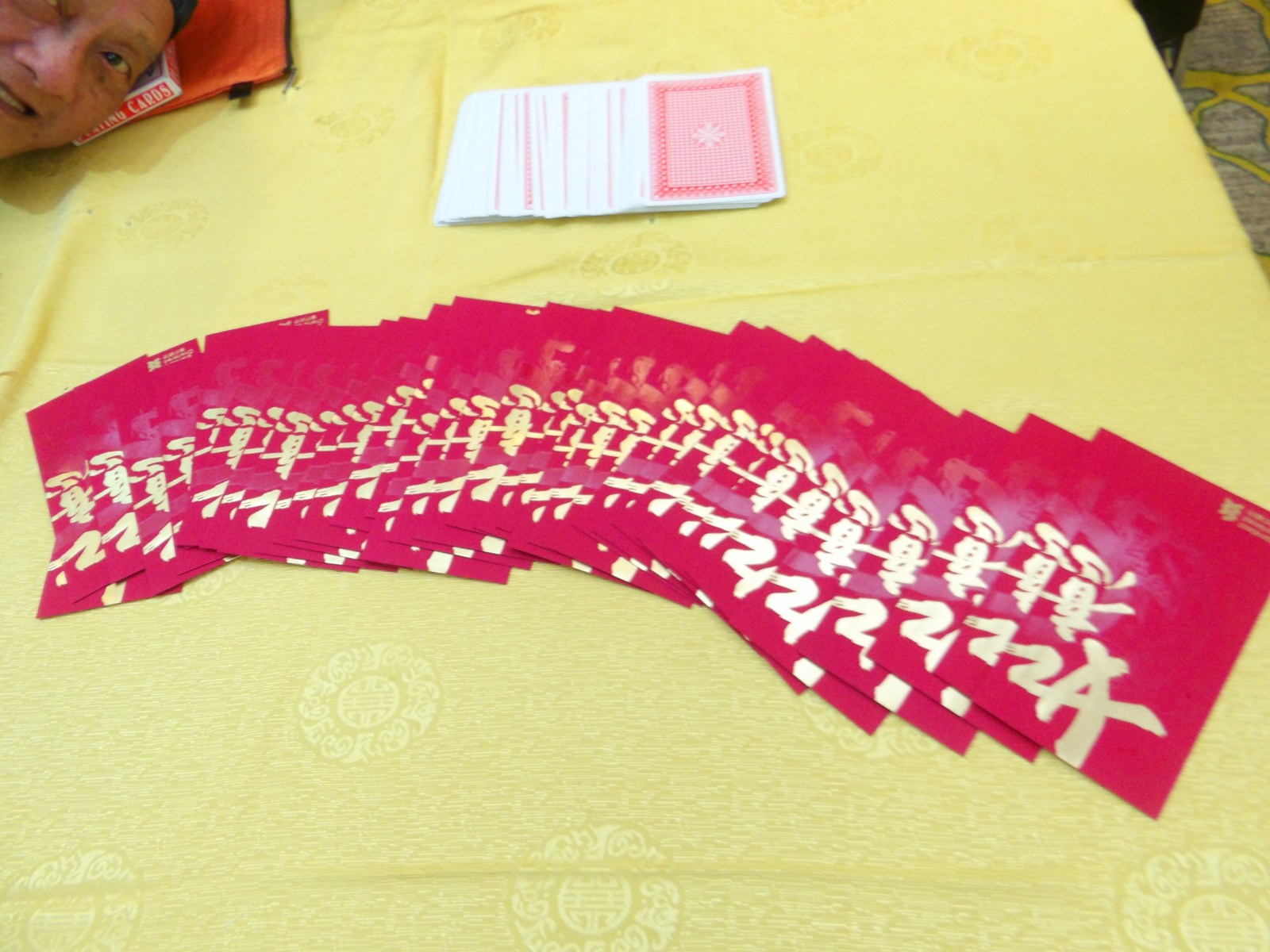This photograph captures a meticulously arranged table with a straight-edged design, adorned by a buttery yellow silk brocade tablecloth, where the folds and creases are prominently visible. At the top of the image, a deck of cards is fanned out face down, hinting at an imminent game or an artistic presentation. Beneath the cards, a series of deep cherry-red pamphlets or envelopes are spread in an elegant arc, each embellished with intricate Chinese script in shimmering gold, adding a touch of cultural richness to the scene. 

In the upper left corner, a man's face can be seen emerging into the frame. His left eye, nose, mouth, and dark hair are visible, suggesting an Asian descent, while his right eye is cut off by the edge of the image. He poses with his head supported on the box from the deck of cards, which is labeled "Playing Cards." Just beneath the deck, an orange zippered envelope with a tab peeks out, possibly a cash envelope.

On the upper right side of the photograph, a hint of a chair is discernible, pushed neatly up to the table. The lower part of the image shows a glimpse of the carpeted floor below, completing a scene that is both intimate and visually engaging.